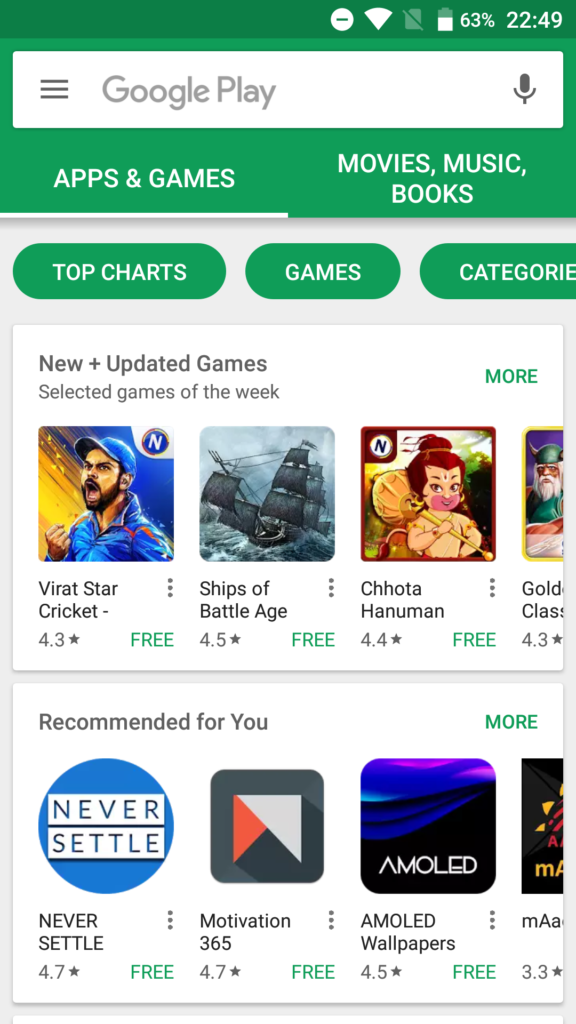This image is a detailed screenshot of the Google Play Store interface on a mobile device. At the top, a dark green status bar displays several icons from left to right: a white circle with a green dash, a white Wi-Fi symbol showing all bars, a gray SIM card icon with a slash indicating no SIM card, and a battery icon that is more than half-filled, showing 63% battery life. The time, displayed in white, reads 22:49.

Beneath the status bar is a lighter green header containing a search bar. On the left, three gray horizontal lines appear on a white background, followed by the text "Google Play" in gray. To the right of this text is a dark gray microphone icon.

Below the header are two tabs. The left tab, labeled "APPS & GAMES" in capital white letters, is selected and highlighted by a bold white underline. The right tab, labeled "MOVIES, MUSIC, BOOKS," is in the same font but not selected.

The section below features a light gray background showcasing three oval icons with green backgrounds and white capitalized text. The icons from left to right read "TOP CHARTS," "GAMES," and "CATEGORIES," though the last icon's text is partially cut off at the end of "CATEGORIES."